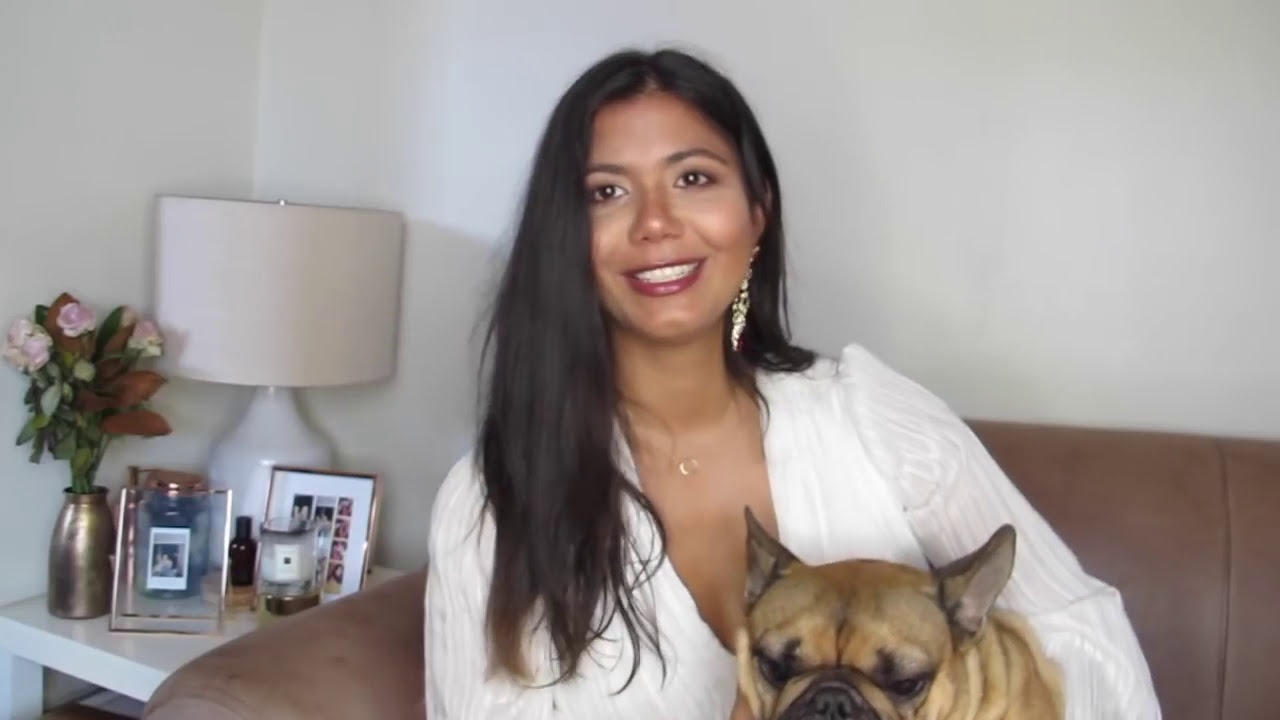In this image, a woman with long, dark brown hair, which is pulled around to the front over her right shoulder, sits on a brown leather couch. She has a tan skin tone and is smiling warmly, showing her teeth. She is wearing a white long-sleeve blouse with a deep plunging v-neck, gold dangly earrings, and a delicate gold necklace. In her arms, she cradles a tan pug, whose ears are slightly back and who faces forward. Behind her, the white wall serves as a backdrop, and to her left on a white side table, there is a white-based, off-white lampshade lamp, a silver vase filled with flowers, two small picture frames—one with a Polaroid and the other with a composite image—and a candle or cup. The setup is cozy and well-lit, capturing a moment filled with warmth and affection.